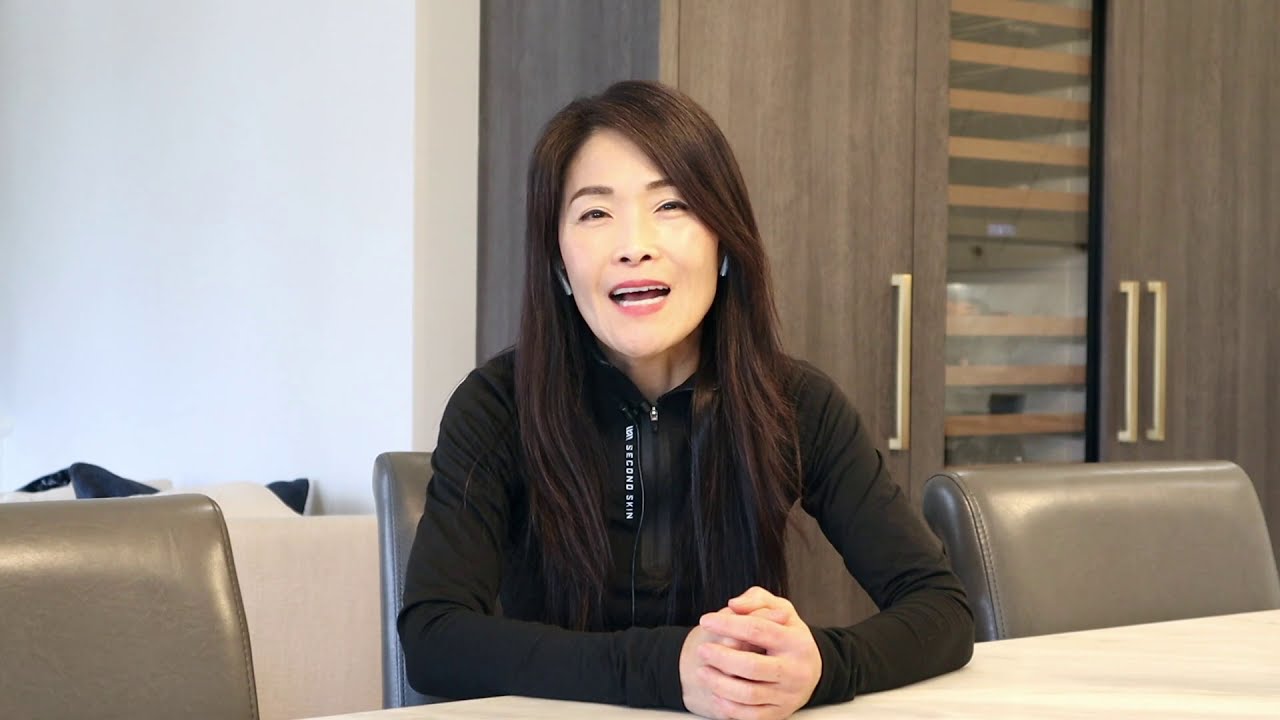The image showcases an Asian woman seated in what appears to be an office or boardroom-like setting. She occupies a gray, plastic or leather chair, positioned in the middle of a long table with adjacent empty seats. The backdrop includes plain white walls, some wooden cabinets with metal handles, and possibly shelving, giving a mixed impression of a workplace or a well-appointed room. The woman, who might be in her 50s but has a youthful appearance possibly due to Botox, has long, flowing black hair that drapes over her modest yet modern black zip-up sweater, which features some small, indistinct text. She wears pink or red lipstick and heavy eyebrow makeup, enhancing her vibrant look. Her expression is caught mid-sentence with an open mouth, likely talking to the camera, suggesting the scene might be part of a photoshoot or video recording for a workplace feature. She appears to wear gray air pods or earrings, and the room's overall ambiance is professional with a touch of warmth.